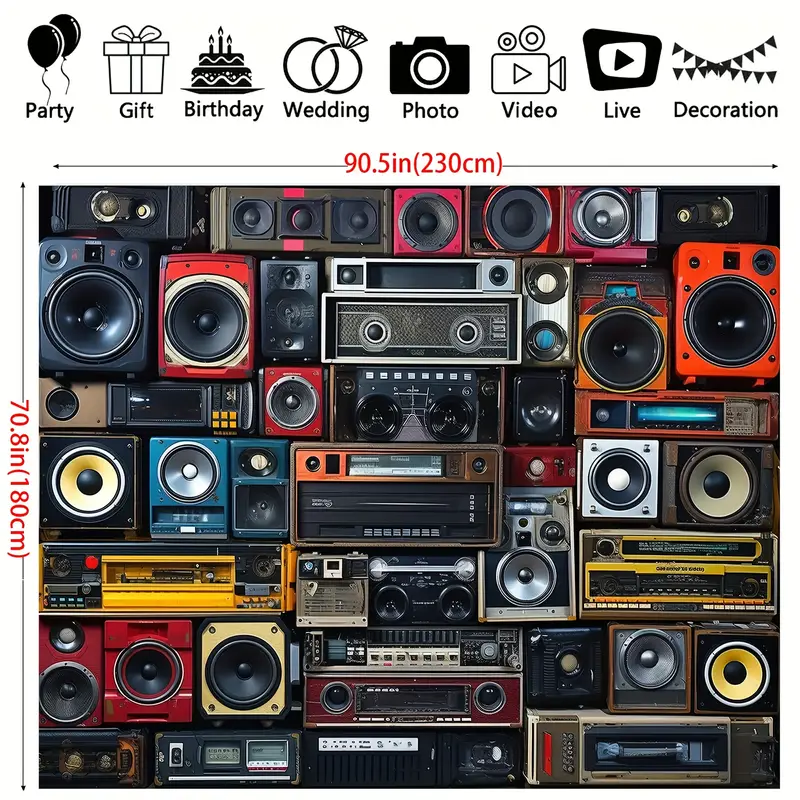The image is a vibrant and eclectic collage of various stereo speakers and audio receivers, overlapping in different shapes and sizes. The speakers come in a variety of colors, including pink, black, red, blue, yellow, and orange. Some speakers are square, while others are rectangular; some stand alone, others are paired, and a few include control dials. The entire collage is framed by dimensions in red text, stating 90.5 inches (230 cm) in width and 70.8 inches (180 cm) in height. Across the top of the image, a horizontal bar features a series of black and white illustrated icons, each accompanied by a descriptive word. From left to right, the icons are: balloons labeled "party," a gift box labeled "gift," a cake labeled "birthday," two rings labeled "wedding," a camera labeled "photo," a camcorder with a play button labeled "video," a rounded play button labeled "live," and a string of triangular flags labeled "decoration." The background of the image is white, as there is no set border or background, giving the collage a floating appearance.